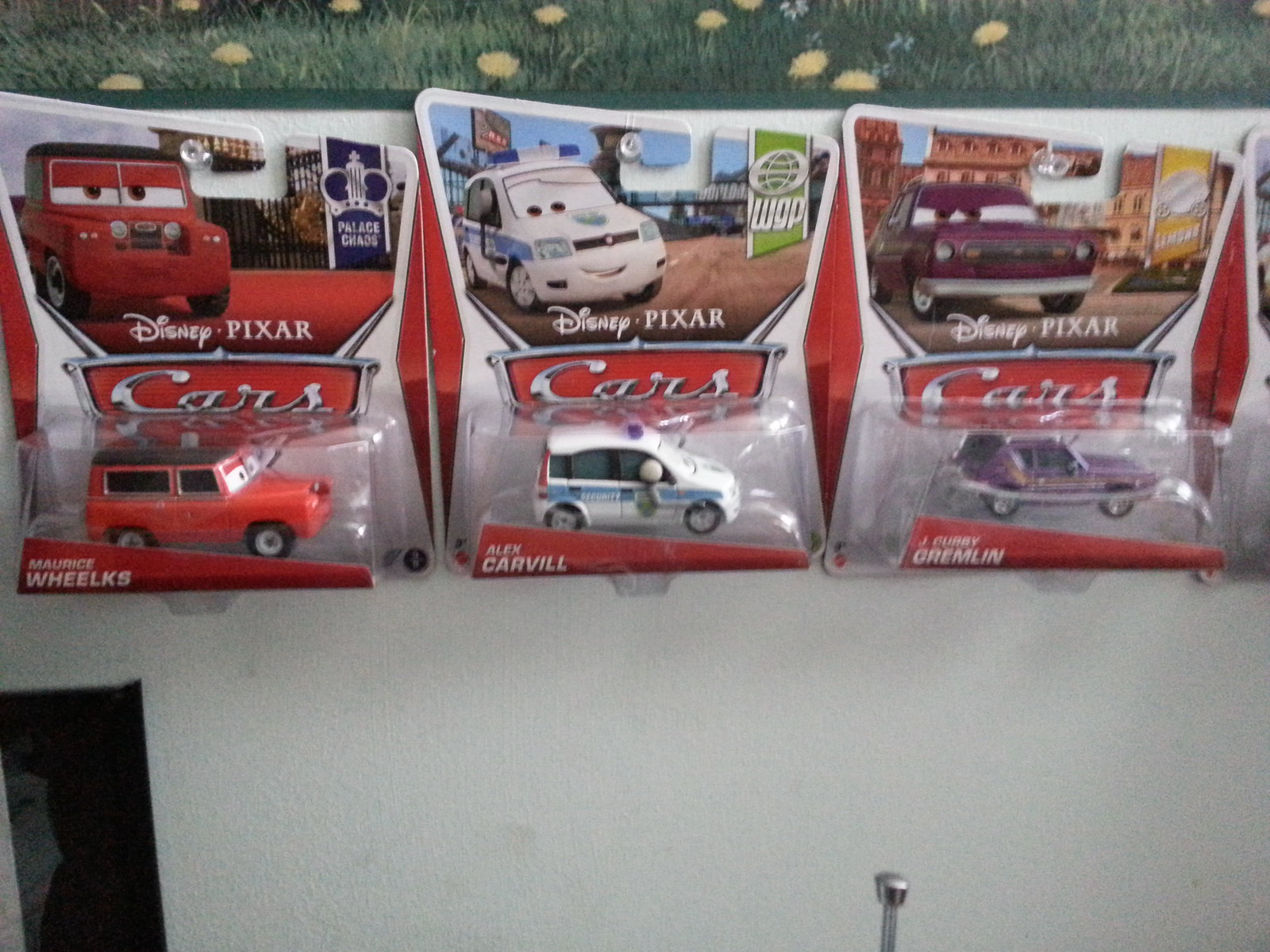This is an outdoor display likely situated at a fair or event, showcasing three packaged miniature cars from the Disney Pixar film "Cars." The display consists of a white shelf with plastic structures that securely hold the items. Each car is encased in a clear plastic bubble attached to a red and white cardboard backing. The packaging prominently features the Disney and Pixar logos in white print, and the word "Cars" is displayed in elegant white script across a red banner. Above each car, there is a large color image of the cartoon character from the movie. 

The three cars are Maurice Welkes, a red SUV-like vehicle; Alex Carville, a white police car; and J. Kirby Gremlin, a purple Gremlin car. The character names are printed at the bottom of each package. The backdrop behind the display is a field of green grass dotted with yellow dandelions. The cars appear to be mounted on the shelf or wall using clear plastic pushpins, visible at the top, adding to the impression that this might not be a typical retail setup. In the background, below the shelf, there is an antenna, suggesting the presence of a radio, which supports the possibility that this is part of a child's collection stored on a wall. The photograph capturing this scene is slightly blurry.